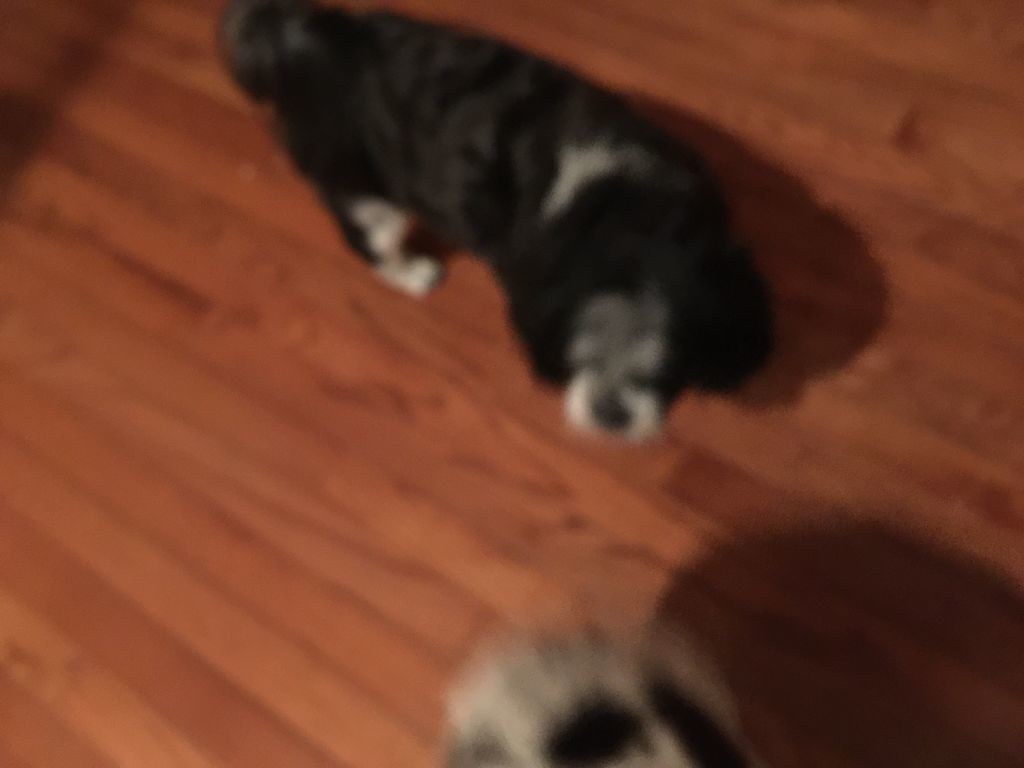A slightly blurry photograph captures a small dog standing on a cherry-colored hardwood floor. The dog appears to be a Lhasa Apso with a recent short haircut, possibly resembling a Cocker Spaniel. Its face is predominantly gray with white markings around the muzzle and eyebrows, while the top of its head and ears are black. A distinctive white stripe is visible across the back of its neck. The dog's body is mostly black, with the exception of its front back legs, which are white. It also has a long, flowing tail. The image is taken from an overhead angle, with the dog looking downward towards the bottom of the picture, where an indistinguishable object or possibly another dog is partially visible.